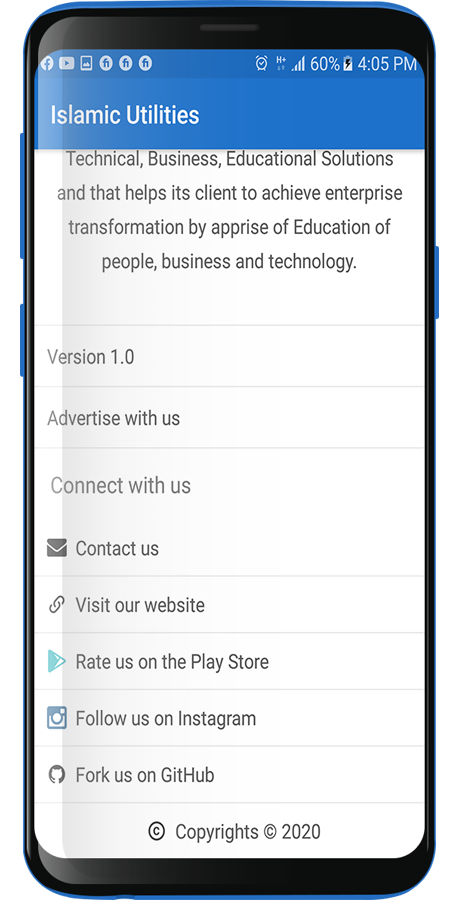In this detailed image, a blue cell phone is prominently displayed, showcasing the "Islamic Utilities" application on its screen. The phone's blue edges and buttons contrast with its black bezel, creating a sleek appearance. At the top left corner, a series of notification icons are visible, including those for Facebook and YouTube. The current time, 4:05 p.m., is shown in the top right corner along with the battery life indicator, displaying 60%.

In the app interface, the top-center features a blue horizontal box with "Islamic Utilities" written in white text. Directly below this, black text on a white background offers a brief description of the app: "Technical, business, educational solutions that help clients achieve enterprise transformation through education in people, business, and technology."

Further down, the app's version is indicated as 1.0. There are several interactive boxes directing users to various sections of the app, such as options to "Advertise with Us" and "Connect with Us." Additionally displayed is a contact link featuring a small mail icon, a link to rate the app on the Play Store highlighted by a teal arrow button, the Google Play Store logo.

At the very bottom of the screen, the copyright symbol accompanied by the text "© 2020" signifies the app's creation and copyright date in the year 2020.